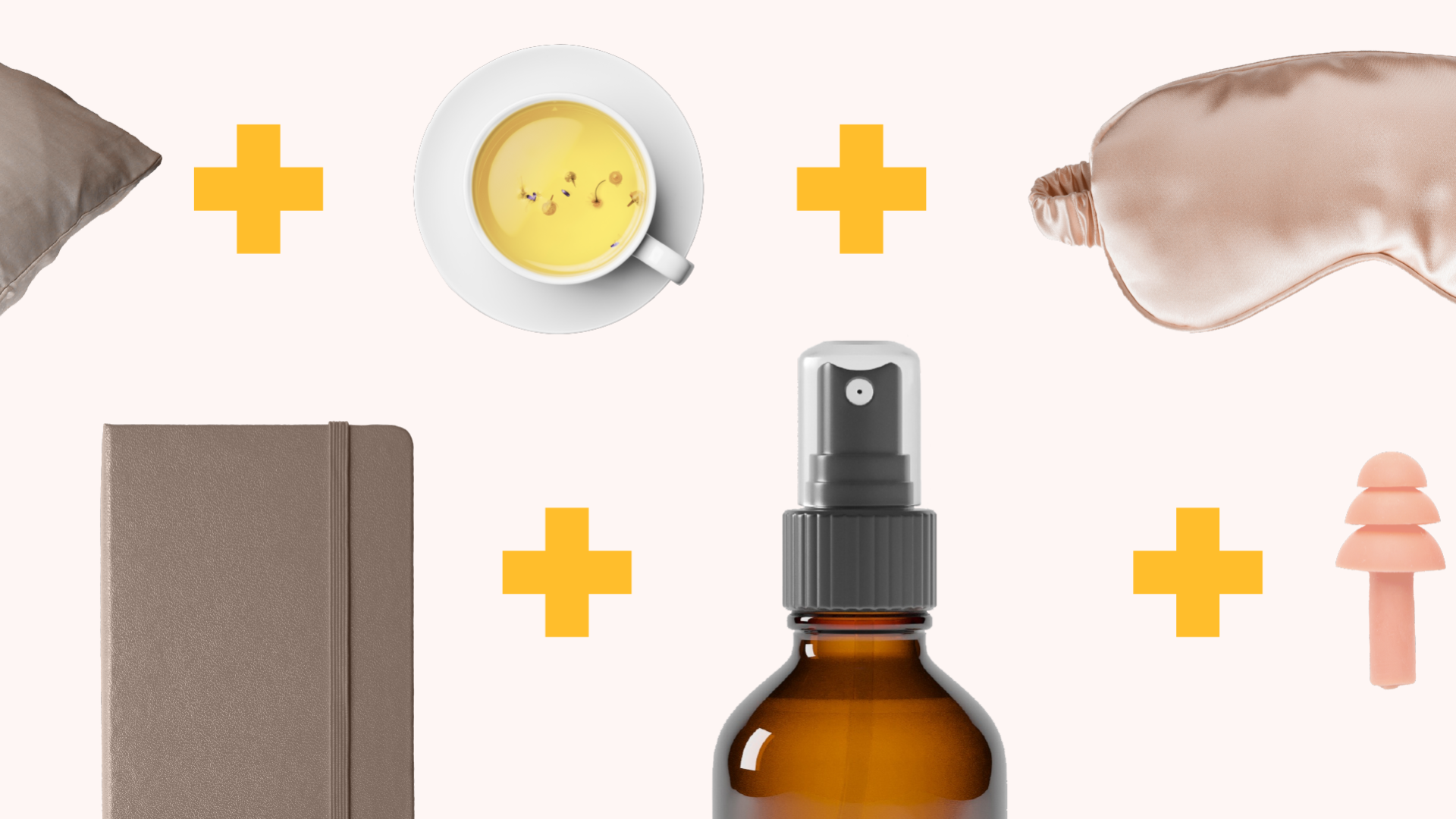The image features a set of diverse items connected by yellow plus signs, arranged in two distinct rows against a soft salmon background. At the top left corner, there's a gray pillow followed by a brown package. Directly to the right of the package is a steaming white teacup filled with yellow herbal tea, set on a white saucer. Adjacent to the teacup is a luxurious, satin pink eye mask.

In the bottom row, starting from the left, sits a gray Moleskine notebook. Moving right, a yellow plus sign leads to a brown spray bottle with a black nozzle and a clear cap. Another yellow plus sign connects this to a set of pink earplugs. The cohesive arrangement of these items and their connections via the bright yellow plus signs seem to suggest a curated set of travel or relaxation essentials, though the exact meaning of their combination remains open to interpretation.